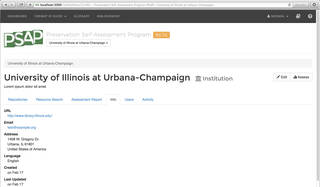The image depicts a low-resolution webpage from the University of Illinois at Urbana-Champaign. The webpage features the acronym "PSAP" prominently displayed in green and white text. The page itself has a relatively small and unclear interface, making it difficult to discern fine details.

At the top of the page, there exists a dark gray banner with several white tabs. Just beneath this area is a search bar set in a grayish interface. To the right of the search bar, there's black text that reads "University of Illinois at Urbana-Champaign," and beside this, the term "Institution" in gray text is visible. Toward the right of this section, there are a couple of buttons, one of which is labeled "edit."

Further down, the page is segmented into various sections delineated by blue tabs and different headlines in black text. Below each headline, various items are listed. Some items are in blue text, including a URL. There are also black text items that provide additional information such as the language "English," a creation date, and other program-related details. The center of the page contains an orange box, followed by a gray text box with black text inside.

Overall, the layout of the webpage includes a series of gray, black, and blue elements interspersed with text that outlines various items and program details.